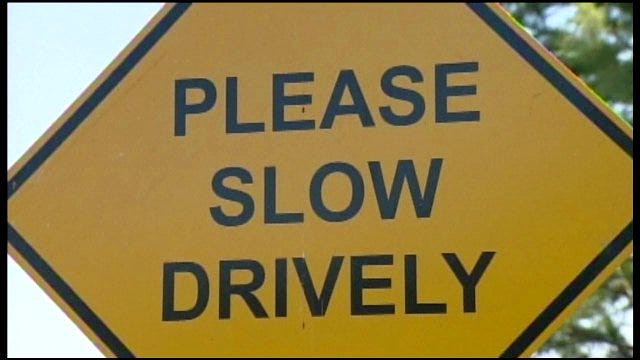A close-up photograph of a yellow sign dominates the image. The sign, appearing to be diamond-shaped, has its top and bottom edges cropped due to the tight zoom. It features a bold, black border and large, capitalized text that reads "PLEASE SLOW DRIVELY." It's unclear if this is a typographical error or if additional letters are simply out of frame. On the left side of the sign, a clear, blue sky is visible, while the right side is framed with green leaves from nearby vegetation, likely trees. The yellow extends slightly beyond the black border, adding a subtle outline to the sign.